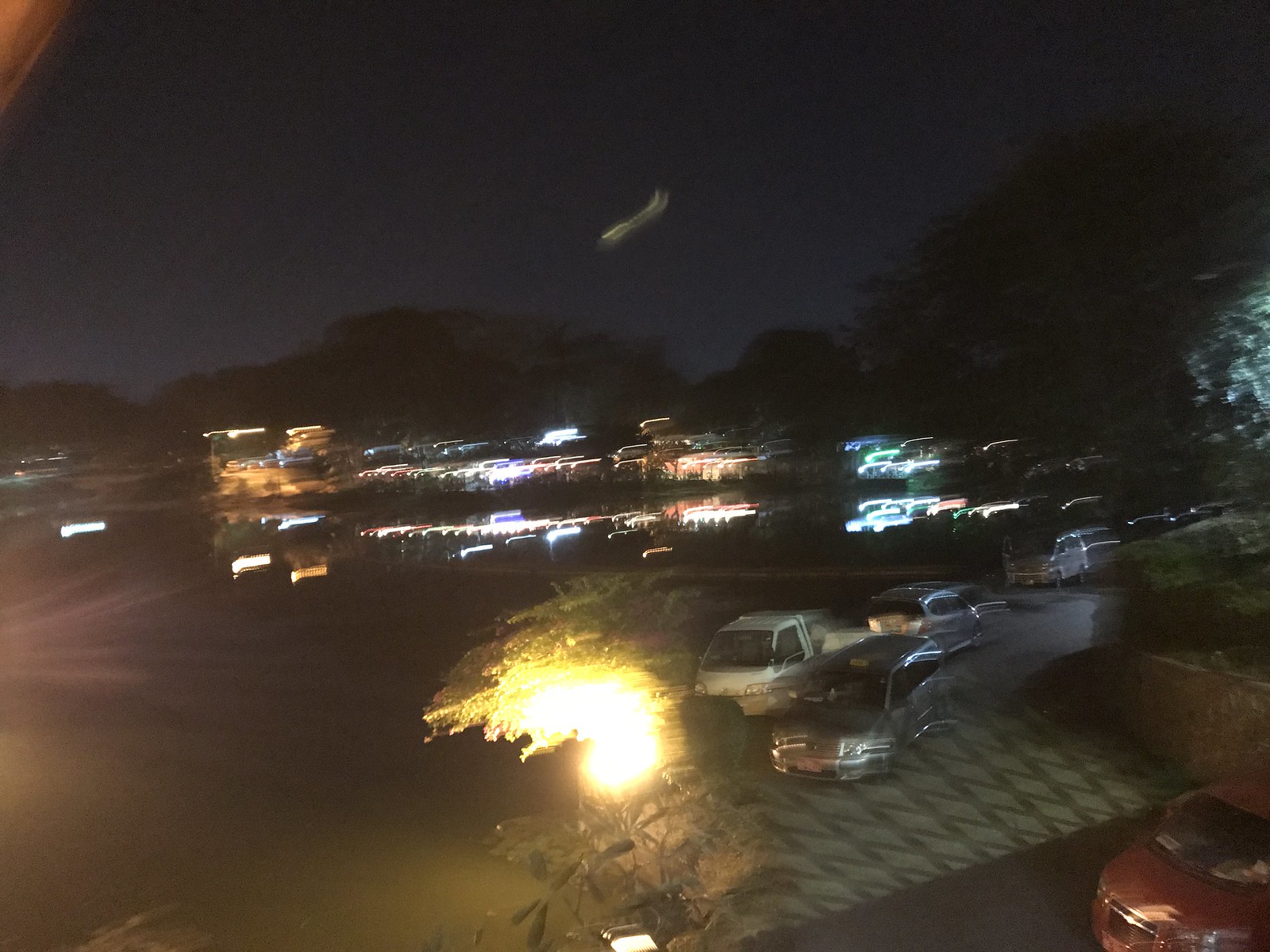This photograph, taken at night, depicts a parking lot in front of a building, possibly a resort or hotel, characterized by significant blurriness and motion blur. The night sky, dark indigo with sporadic clouds, forms the backdrop above a horizon lined with tall trees and shrubs. In the shot's foreground, there's a mix of faint light sources, likely from streetlights and nearby buildings, creating a tapestry of blurry lights. On the right-hand side, a streetlight illuminates a tree, casting an eerie glow. The parking lot hosts several cars: a red car at the front, followed by a gray SUV, a white car, and another gray car with its trunk open. Additionally, there's a small truck and other vaguely visible vehicles. At the bottom center of the image, a tree or shrub appears to glow, possibly from a nearby light. The overall composition includes a gray road, a ledge with a green bush on the right side, and distant green trees. The upper portion of the image showcases the blue night sky with two wavy white lines, enhancing the impression of a late evening scene.